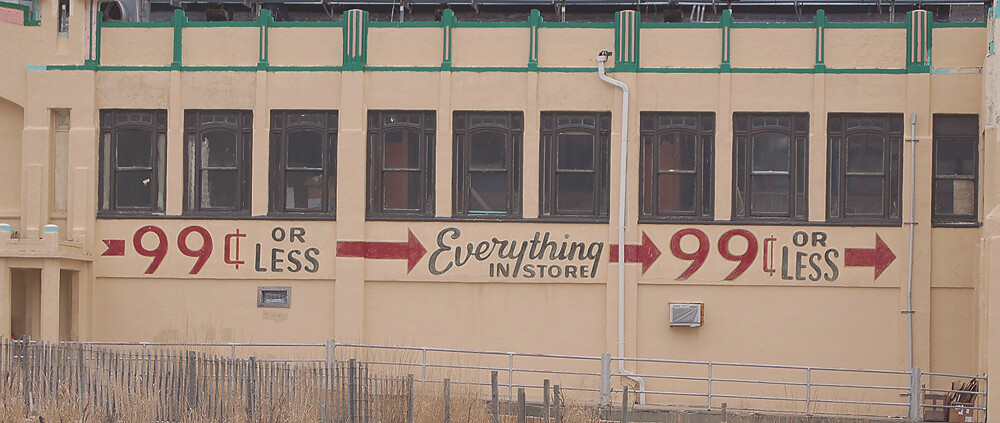In this high-quality photograph, the foreground features a metal fence partially obscuring a tan-colored building with green detailing near the roofline. A row of dark windows is lined up just below the green accents. Prominently displayed beneath the windows is signage with a mix of red and black text: "Everything in Store $0.99 or less" accompanied by several red arrows pointing downward. To one side, an air conditioning unit covered in plastic is visible, and alongside it runs a white drainpipe extending vertically down the building. On the opposite side, a silvery grate adds to the urban texture of the scene. The building's facade shows slight signs of wear, with noticeable dirt along parts of its exterior.